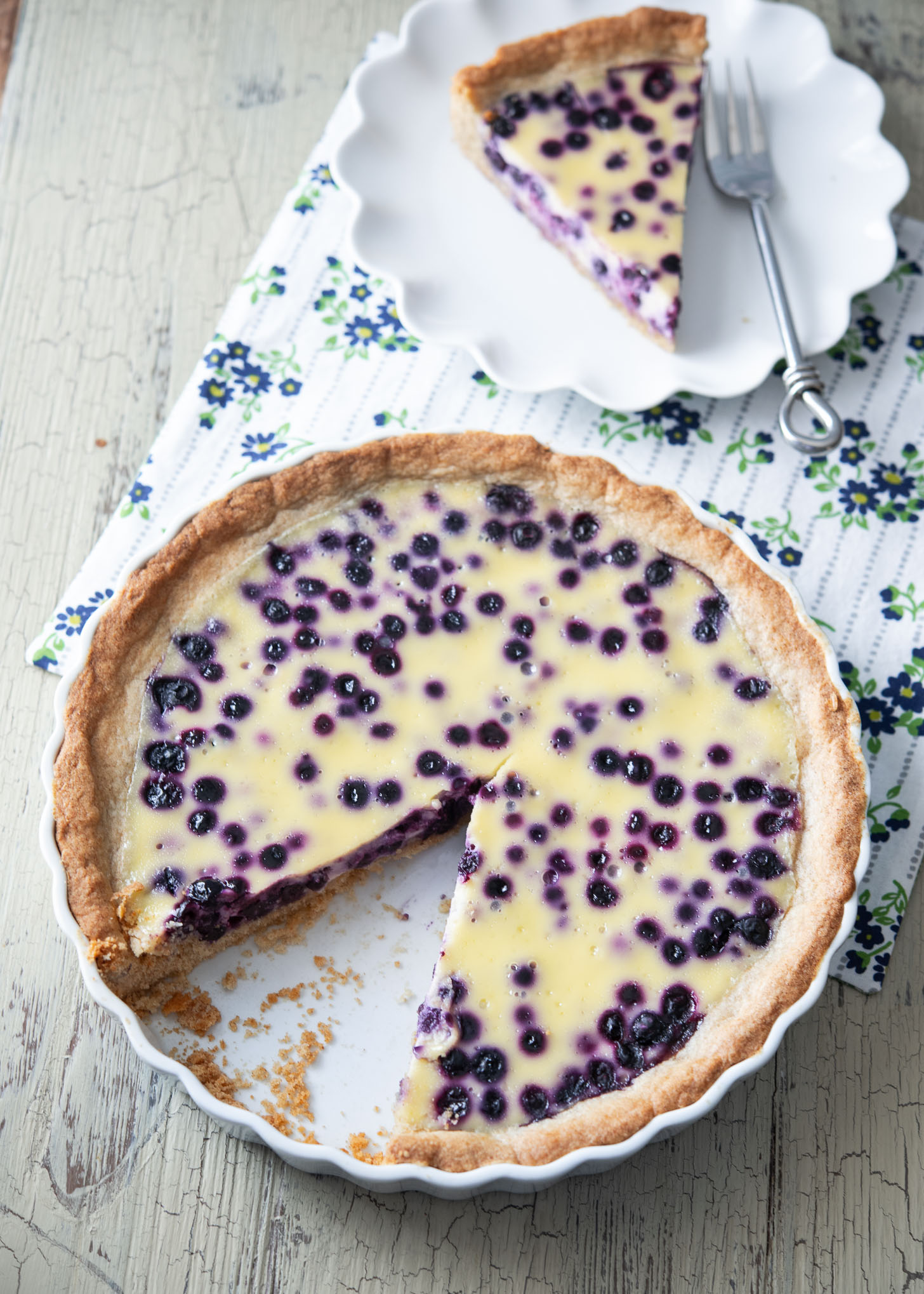The outdoor photograph captures a rectangular scene featuring a homemade blueberry custard pie. The pie, seated in a white circular pie dish, occupies the bottom half of the image. Its rich blend of creamy white custard layers topped with plump blueberries can be seen throughout. A triangular slice has been meticulously cut and placed on a white scalloped saucer, accompanied by a silver fork. Both the pie dish and saucer rest on a worn, grainy white wooden table, partially covered by a white fabric place mat adorned with delicate blue and yellow floral patterns. Subtle shades of brown, cream, purple, silver, blue, yellow, and green add to the overall rustic and inviting ambiance of the scene.